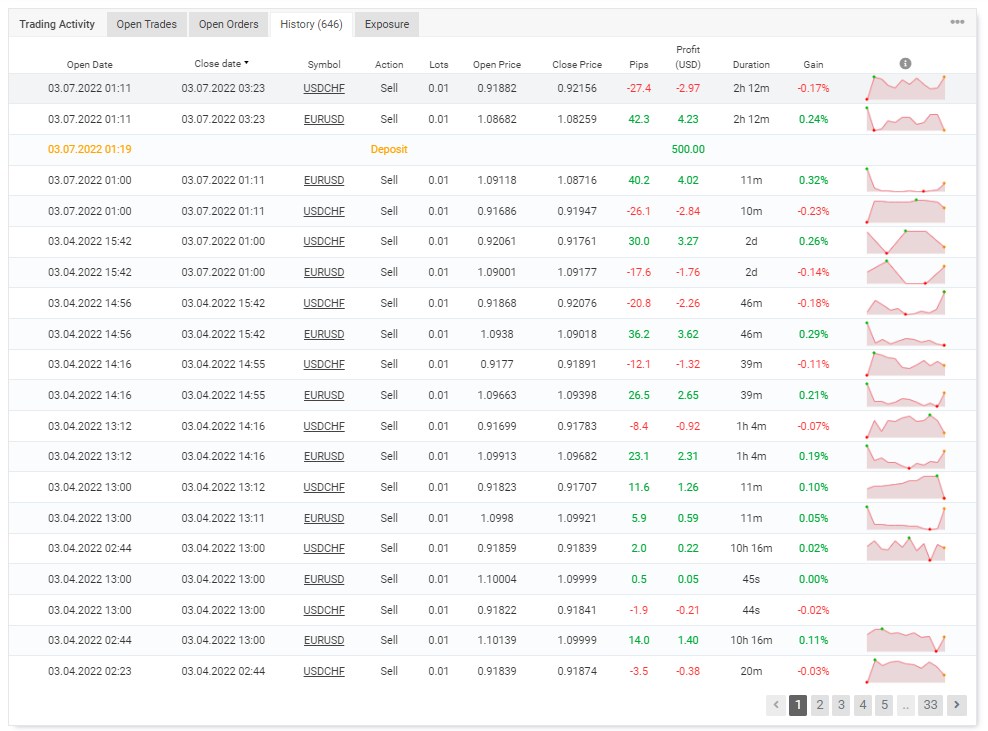This image is a detailed screenshot of the MetaTrader app, showcasing a user's personal trading history on the platform. The interface is divided into several tabs at the top: Trading Activity, Open Trades, Open Orders, History, and Exposure. The 'History' tab is selected, displaying a comprehensive account of the user's past trades.

At the top of the history section, there are multiple columns categorized under various headers: Open Date, Close Date, Symbol, Action, Lots, Open Price, Closed Price, Pips, Profit, Duration, Gain, and Performance Graphs. Each column contains a vertical list corresponding to its header, detailing the specifics of each trade made by the user. 

The 'Open Date' column lists the initiation dates of trades, while the 'Close Date' column records when those trades were concluded. The 'Symbol' column identifies the traded assets, and the 'Action' column indicates whether the trade was a buy or sell. 'Lots' specifies the trade volume. The 'Open Price' and 'Close Price' sections display the starting and ending prices of the trades, respectively. The 'Pips' column shows the movement in price, while 'Profit' delineates the financial outcome of each trade. 'Duration' marks how long each trade was held, followed by 'Gain' which highlights any increases or decreases in value. At the far right, small line graphs provide a visual representation of the performance of each trade.

At the bottom right of the screen, there is a pagination control with numbered boxes and left and right arrows. The number '1' is currently selected, indicating that the view is on the first page of the user's trading history.